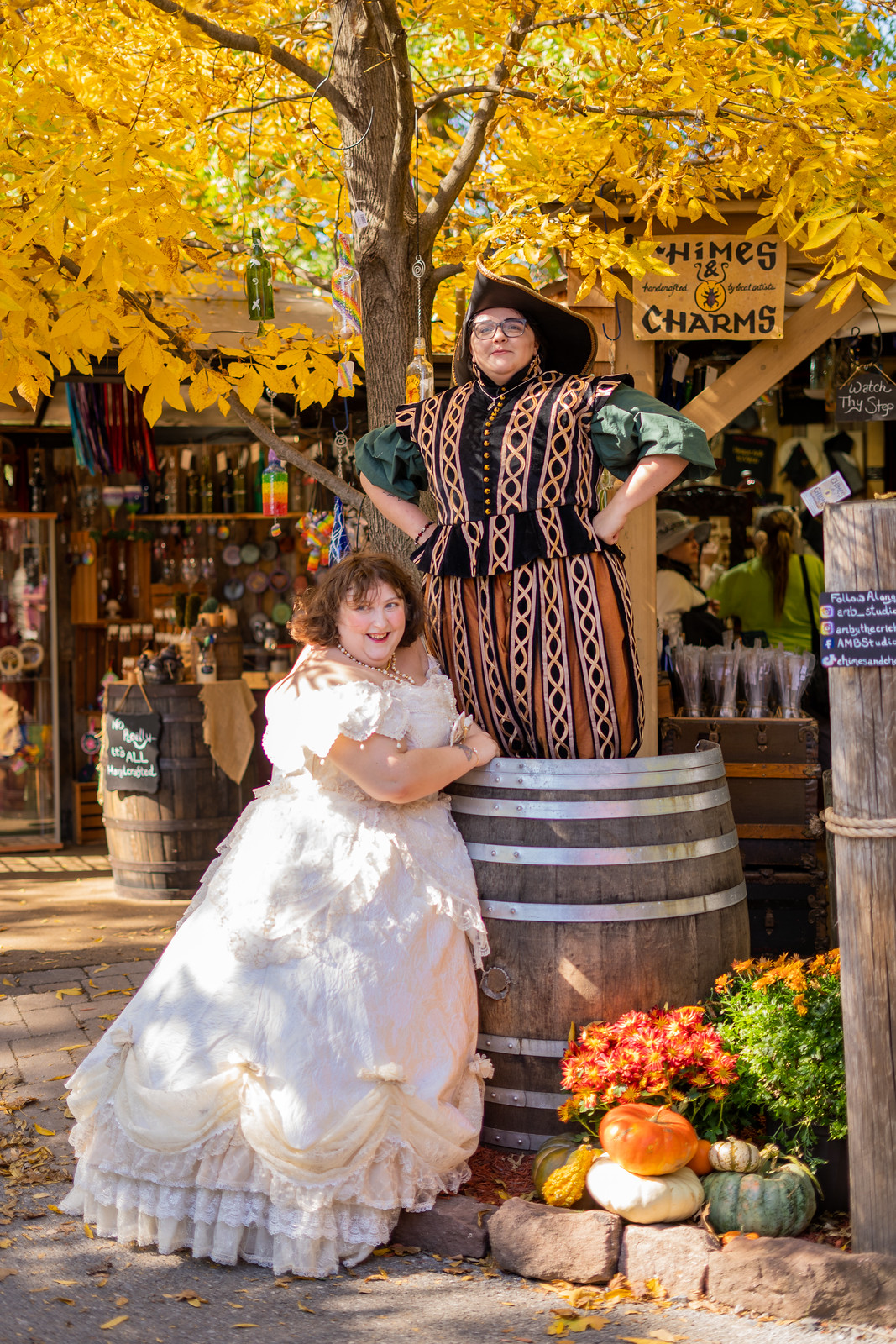The image portrays a vibrant scene reminiscent of a festive medieval event. Two women are the focal point in this portrait-oriented photograph. One woman is standing inside a barrel, visible from the knee up. She is dressed in a jester-like outfit featuring orange, green, and gold colors, and she accessorizes with a sizable black pirate’s hat and glasses. Her hands rest confidently on her hips. Leaning on the barrel beside her is another woman adorned in a voluminous white dress, her brown hair framing her smiling face.

The background cascades with the yellow hues of fall leaves from nearby trees, setting an autumnal mood. In the foreground, pumpkins and various boards suggest a festive setting. A bit of brick and concrete road is also visible. Further back, a storefront comes into view, displaying bottles, signs, and additional barrels, indicating perhaps a festival marketplace. The scene is filled with details of a historical reenactment or themed celebration, blending the charm of medieval aesthetics with the vibrancy of a seasonal fair.